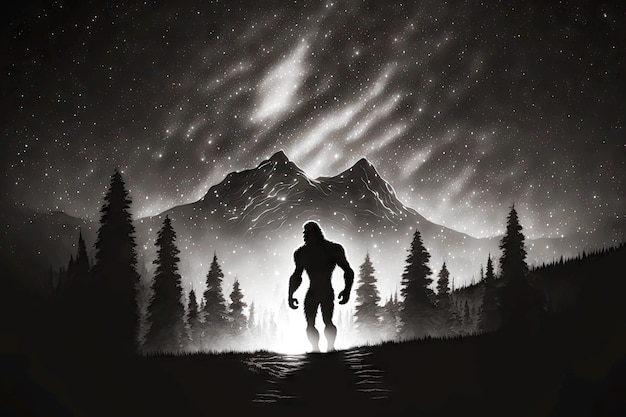This black and white, hand-drawn illustration captures a mysterious nighttime landscape. Central to the scene is a large, humanoid figure resembling Bigfoot, standing prominently in silhouette. The creature, with its broad shoulders, long, muscular limbs, and fur-covered body, is enveloped in an eerie, white aura, highlighting its presence in the dark setting. Situated within a valley, it faces slightly right, with its distinct profile visible against the well-lit mountain range featuring twin peaks.

Surrounding the central figure, tall conifer trees line a path that cuts through the lower center of the image, creating a dense forest atmosphere. The ground is subtly dotted with small patches of snow, adding to the wintery feel, though it melds with the darkness of the terrain. The sky above is a dramatic mix of black overhead with bright, starry clouds and constellations that light up the horizon and mountains, giving the impression of an aurora borealis effect. This ethereal backdrop, combined with the stark contrasts and detailed landscape featuring hills and pine trees on either side, enhances the enigmatic and almost mythical presence of the creature in this rural, nighttime scene.